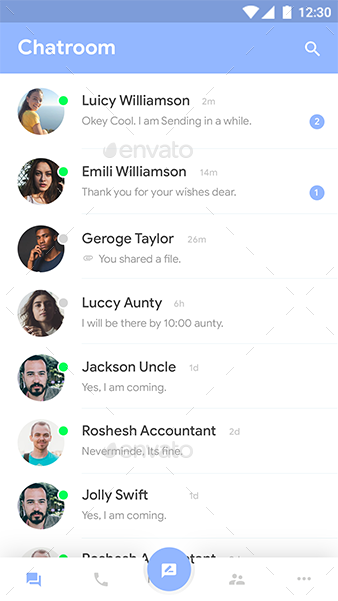This is a detailed mobile screenshot featuring a chat room interface. At the top, there's a thin blue banner followed by a light blue banner beneath it, against a white background. A watermark from Envato spans diagonally across the image. In the upper left corner, the "Chat Room" title is displayed, accompanied by three icons, the time "12:30," and a search icon.

The main section presents a list of people in the chat room with profile pictures on the left side of their names. The list includes the following users from top to bottom: Lucy Williamson, Emily Williamson, George Taylor, Lukey Onty, Jackson Uncle, Roshish Accountant, and Jolly Swift. Each name has a small green dot next to their profile picture, indicating they are online, with the exception of George Taylor and Lukey Onty. Each user's name is also accompanied by a brief status message or saying.

At the bottom of the image, five icons are present in a footer bar. The central icon is obscured by a blue circle and a text box. An additional user is partially visible but cut off by the footer bar. The watermark, blue banners, and dotted diagonal line are consistent elements throughout the image.